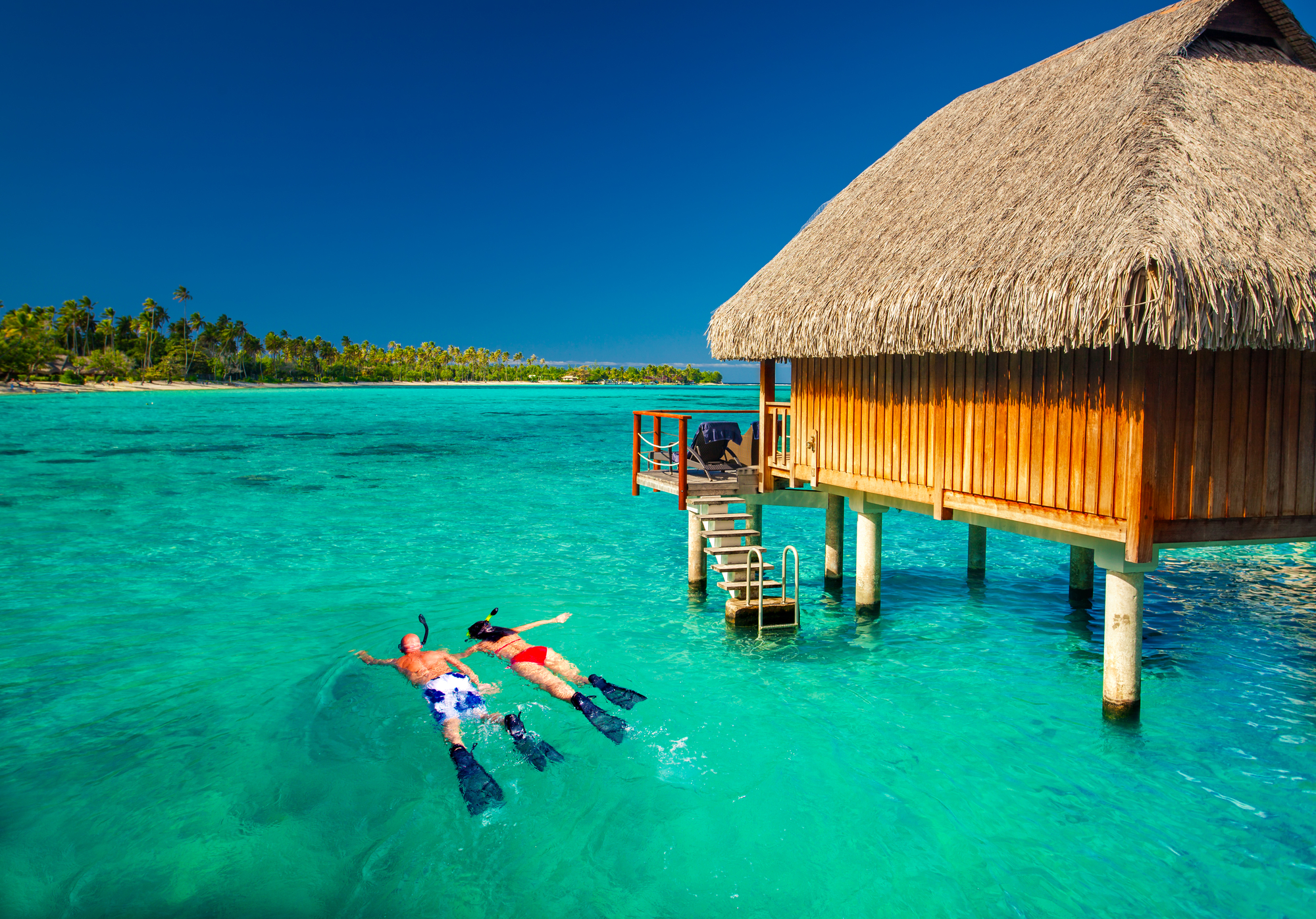This stunning vacation scene showcases a serene and idyllic waterscape, reminiscent of the French Polynesian paradise of Bora Bora. In the foreground, two fit individuals are snorkeling in crystal-clear green-blue seawater. The man, bald and tan, is wearing blue and white trunks with black fins, while the woman, with dark hair, dons a red bikini and blue fins. Both have snorkels protruding from the water as they float face down, exploring the underwater beauty.

To their right, a charming reed-style and wooden hut on large round wooden pillars is suspended above the water. This hut features a thatched roof and wood sides, complete with a set of steps leading out of the water to a small deck, where a balcony with chairs invites relaxation and scenic views. The water around them is smooth and teeming with vibrant oceanic life.

In the background, a sandbar adorned with lush green palm trees stretches out, enhancing the tropical allure of the scene. The sky above is a flawless, deep blue, completing this picturesque snapshot of paradise.